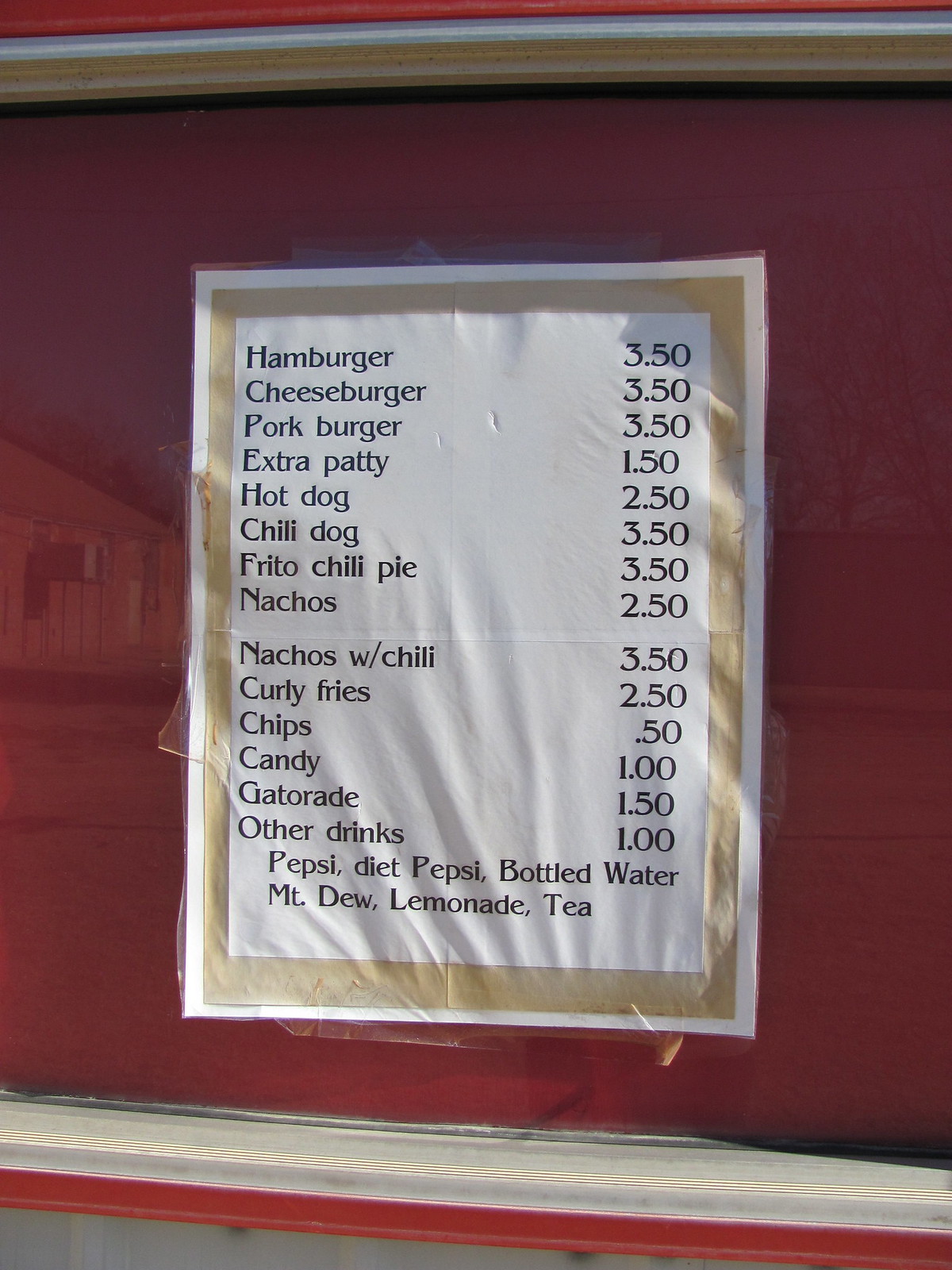This image captures a worn menu from a food truck or possibly an outdoor food stand. The menu, printed on a white laminated sheet, is taped to a red background, which could be the side of a food truck or a wall. A creamish-tan border frames the menu, showing signs of age with visible crinkles and creases, suggesting it has been in place for some time. Above and below the menu, horizontal lines hint at a structure, possibly indicating the presence of a window that opens for food service.

The offerings are neatly listed from top to bottom as follows:
- Hamburger: $3.50
- Cheeseburger: $3.50
- Pork Burger: $3.50
- Extra Patty: $1.50
- Hot Dog: $2.50
- Chili Dog: $3.50
- Frito Chili Pie: $3.50
- Nachos: $2.50
- Nachos with Chili: $3.50
- Curly Fries: $2.50
- Chips: $0.50
- Candy: $1.00
- Gatorade: $1.50
- Other Drinks: $1.00, which includes Pepsi, Diet Pepsi, Bottled Water, Mountain Dew, Lemonade, and Tea.

The descriptive nature of the menu and its detailed items suggest a straightforward, no-frills dining experience, characteristic of casual food truck fare.